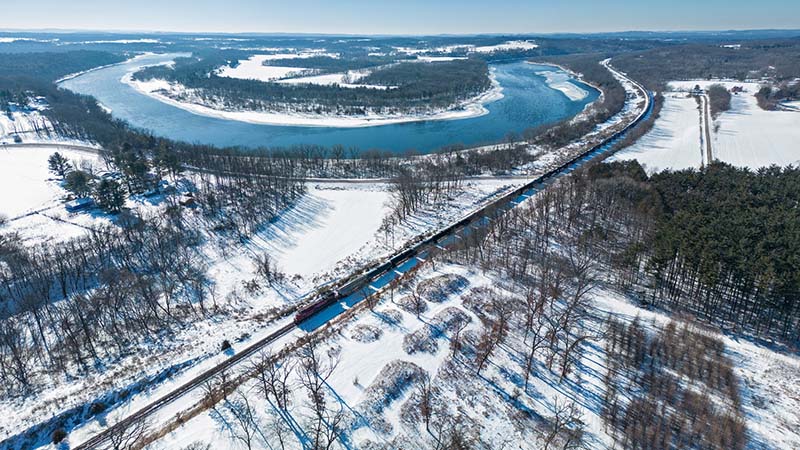The photograph is an aerial view of a vast, snow-covered landscape, capturing a full-color, rectangular image where the horizontal edge is the longest. Dominating the scene is a long train winding through the snowy terrain. The train tracks cut diagonally from the middle of the image, curving down towards the bottom left. To the right, there is a dense forested area, while sparser trees, leafless and dusted with snow, are visible on the left. Above the train, a striking blue river weaves in an oxbow-like formation, encircling a small piece of land connected to the main landmass, resembling a peninsula. The overcast sky is a grayish blue, contributing to the wintry atmosphere that blankets the entire river and landscape with snow. The scene is devoid of any text or artificial elements, focusing purely on the natural beauty and stark contrast of the snow-covered environment against the flowing blue river and winding train tracks.